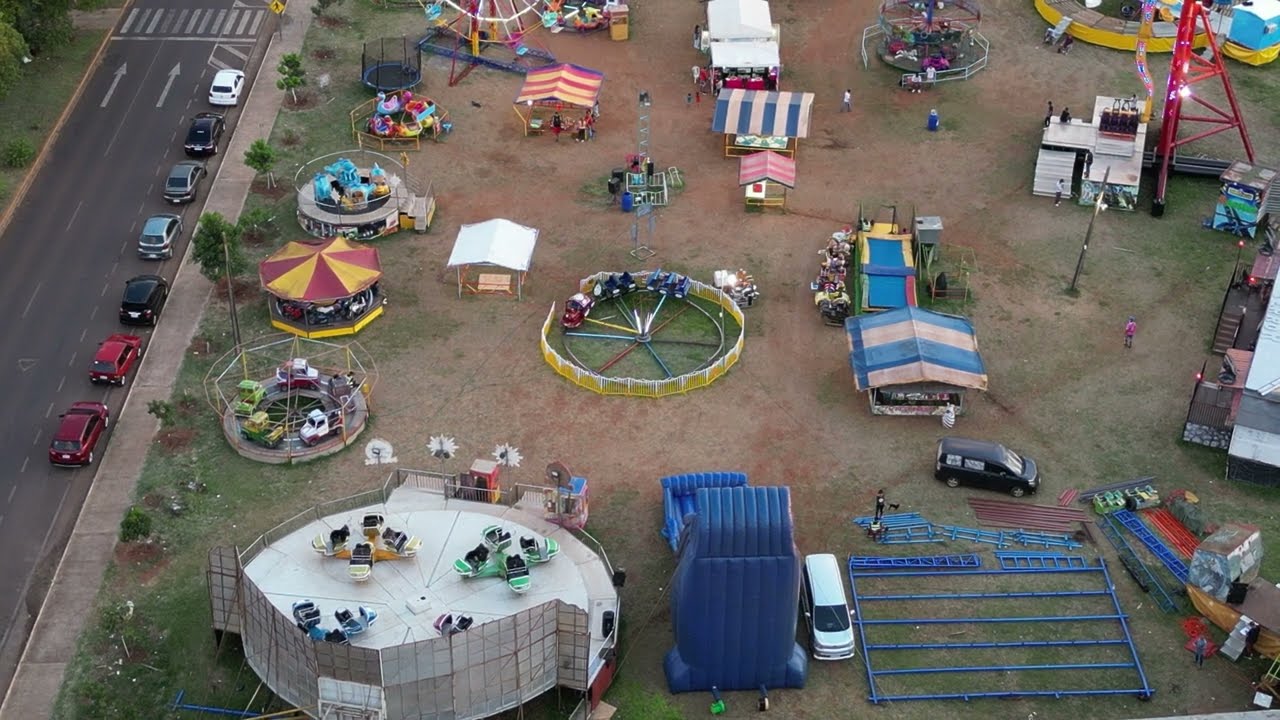This detailed overhead shot captures a bustling carnival set up in a large dirt patch interspersed with worn grass patches. Central to the scene are numerous carnival rides and small attractions, including a ferris wheel nestled in the back left of the image, a merry-go-round, a spinning cars ride, and possibly a tilt-a-whirl. Several rides and game stands cater specifically to children, with four smaller attractions lined up next to a sidewalk on the left side. The food and concession stands are distinguishable by their striped, triangular-shaped roofs in various colors: blue and white, white and grey, and red and yellow. The carnival is bordered by a sidewalk, beyond which a street is visible, lined with about seven parked cars. Adding to the urban atmosphere, there are three lanes of traffic visible to the left. On the lower right, there is a small stage or concert venue, and metallic-looking pieces, blue in color, are being set up, with a man actively working on them, indicating ongoing preparations.